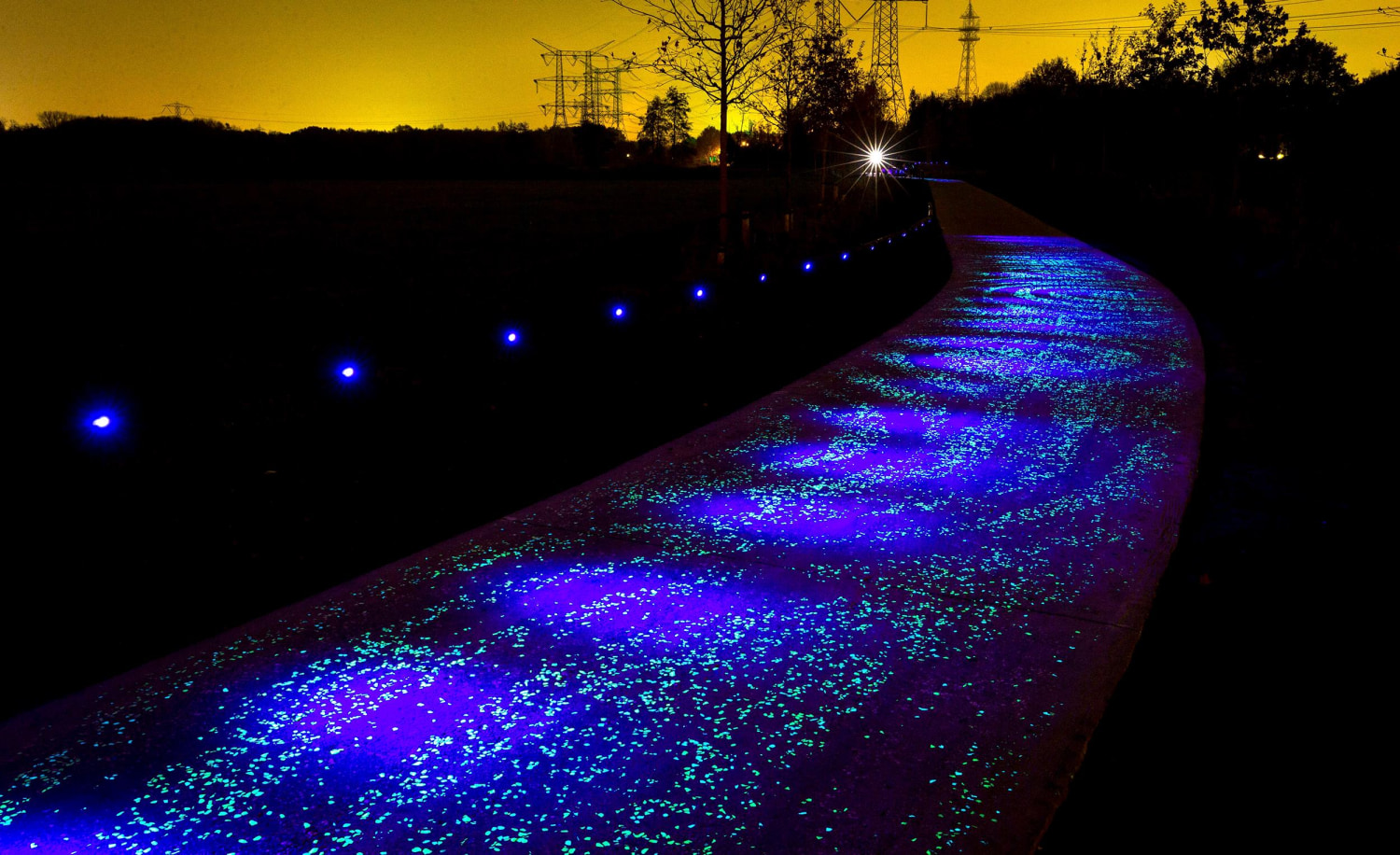This nighttime twilight photograph captures an enigmatic pathway winding off into the distance under a glowing dim yellow horizon. We're positioned on this colorful sidewalk, which is vividly illuminated by intense black lights. The path itself is painted with a mesmerizing combination of fluorescent purple and green speckled paint, glowing brightly amid the darkness. These small but intense black lights are placed along the sides of the walkway, emphasizing the neon patterns adorning the path.

As the pathway extends away, it twists from the lower left corner of the image and meanders towards the upper right, fading into the horizon. The sky at the horizon glows a dim yellow, adding to the surreal ambiance of the scene. Tall power lines and girded tension supports are silhouetted against this faint light, punctuating the horizon and adding to the scene's depth and structure. On either side of the path, darkness prevails, enveloping everything except the lit pathway and its adornments with an impenetrable blackness.

While the scene appears to be a photograph, the vividness of the colors and the perfectly placed lighting suggest potential digital enhancements, adding a possibly computer-generated quality to the image. The intense, glowing paint, and evenly spaced black lights create a surreal, almost otherworldly feel to this otherwise tranquil moment captured at twilight.